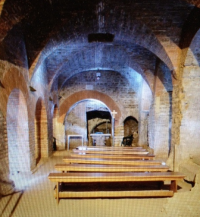This blurry, small, square image likely depicts the interior of a church or catacombs, characterized by its brick or stone walls and multiple arches. The room, which appears dimly lit, features a dark overhead ceiling with bright light filtering in through the arches. At the front of the room, there is a prominent cross and a white altar or statue, illuminated by a brighter light. The floor is tan, and there are six modern wooden pews arranged in rows, though no people are visible in the image. The overall atmosphere is quiet and solemn, enhanced by the empty benches and the lack of additional decor or writing on the walls.